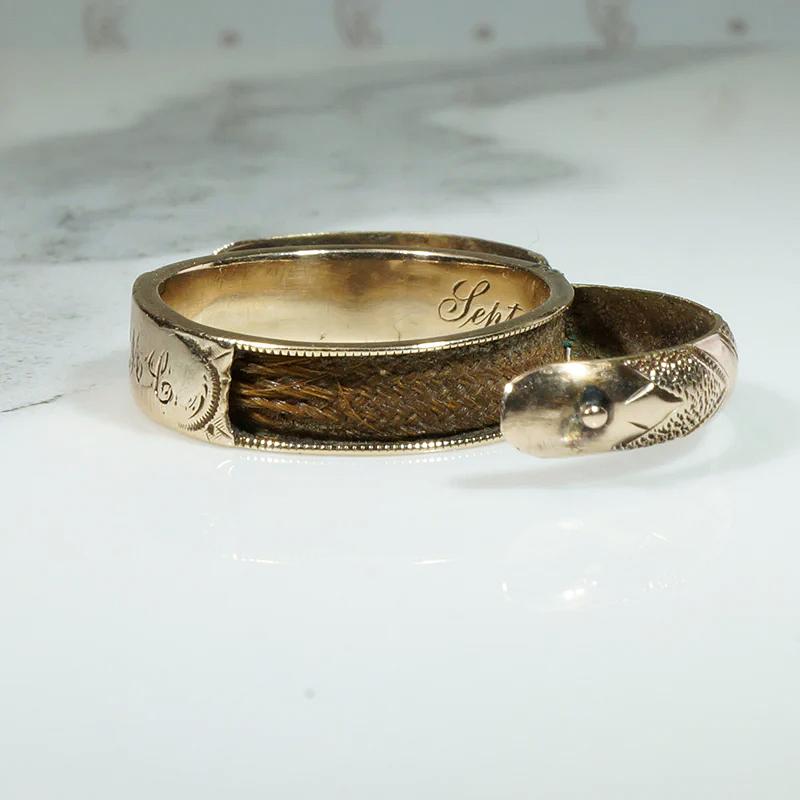This photograph showcases a piece of antique jewelry, elegantly displayed on a slightly off-white, ceramic or marble countertop. The central feature appears to be a golden ring or bangle bracelet, distinguished by its intricate design. The jewelry exhibits a woven texture reminiscent of a snake's body, where the gold covers half of the braided pattern before transitioning into a snake head motif. Part of the piece appears to be unclasped or pulled out, exposing a brown, waxy inner texture that enhances its aged, slightly tarnished appearance.

Both the inside and outside surfaces of the jewelry bear cursive engravings. A small, gold circle at the center features an inscription that is challenging to decipher but seems to read "L-E-H-T" or "J-E-H-T." Additionally, another section inscribed with "S-E-P-T" could be identified amidst the ornate design. The overall impression is one of an antique, possibly handcrafted item, detailed with fine engravings and a unique, symbolic design.